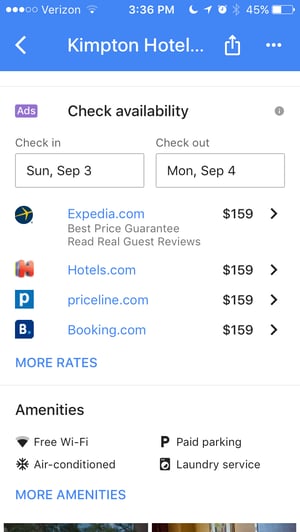A detailed screen capture from a Verizon user's cell phone at 3:36 PM shows a 45% battery charge with three bars of signal strength and very weak Wi-Fi. The screen displays a page for "Kempton Hotel," including a section labeled "ads." The user is looking at hotel availability, with check-in set for Sunday, September 3rd, and check-out for Monday, September 4th. Pricing quotes from four different travel sites—Expedia, Hotels.com, Priceline.com, and Booking.com—each list a rate of $159 for the selected dates. Below the pricing information, the amenities are listed: free Wi-Fi, air conditioning, paid parking, and laundry service. As the page is scrolled down, there is a "More Amenities" section that starts to reveal the tops of some photographs, indicating additional images are available for viewing.